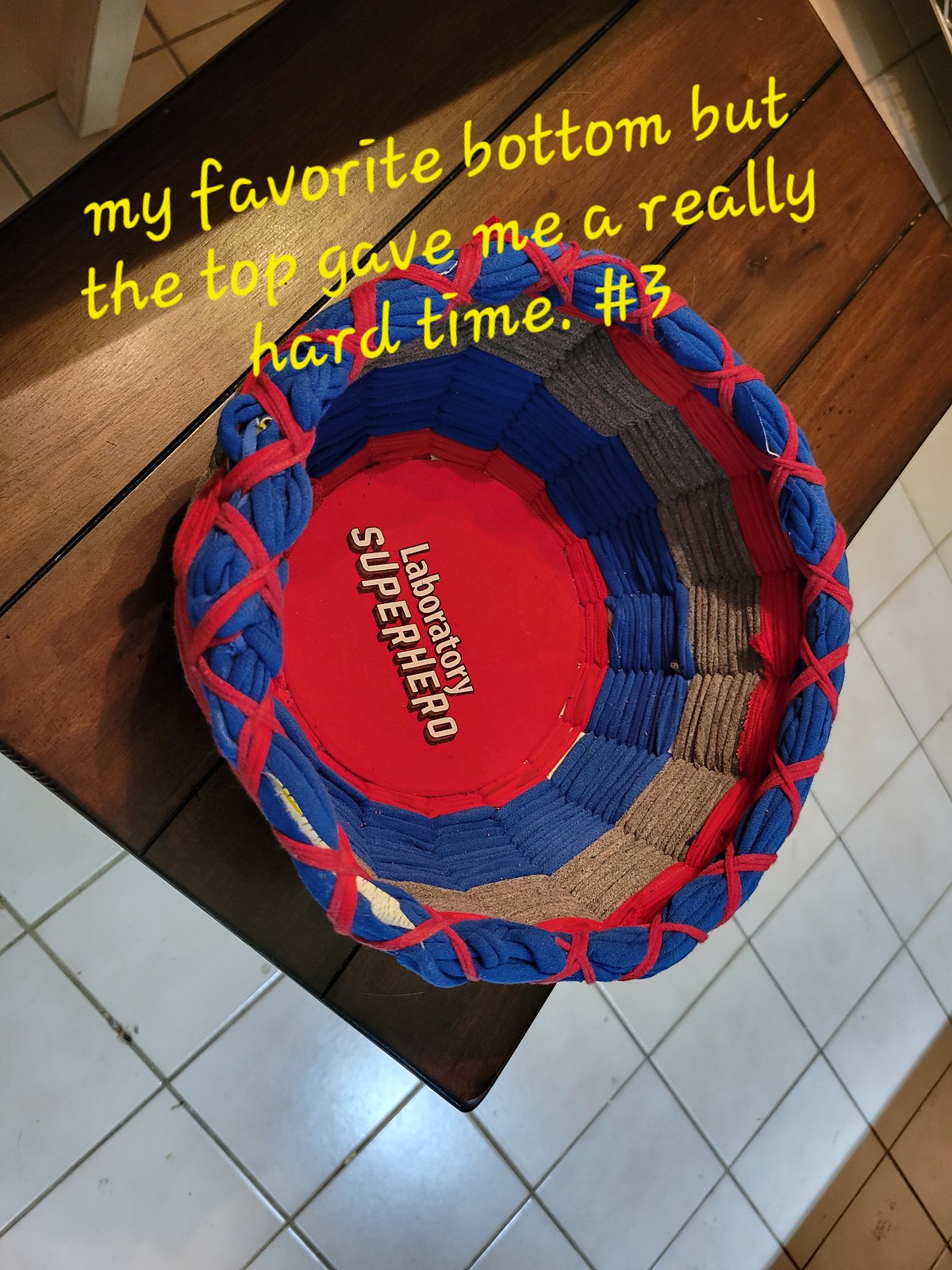The image features a vibrant, handmade woven basket crafted from cloth rags, yarn, and possibly discarded fabric strips. This circular basket showcases an array of colors, including a red base, followed by layers of blue, gray, and more red, culminating in a blue top adorned with red cross-stitched X's. A red circular patch at the bottom interior of the basket reads "Laboratory Superhero." The image is slightly angled, revealing a dark brown, four-slat wooden board upon which the basket stands, set against a white tile floor. In the upper part of the photo, there is yellow text, slightly offset to the left, that reads, "My favorite bottom, but the top gave me a really hard time, #3." The woodgrain background and evident smudge marks on the tiles below add a rustic feel to the scene.